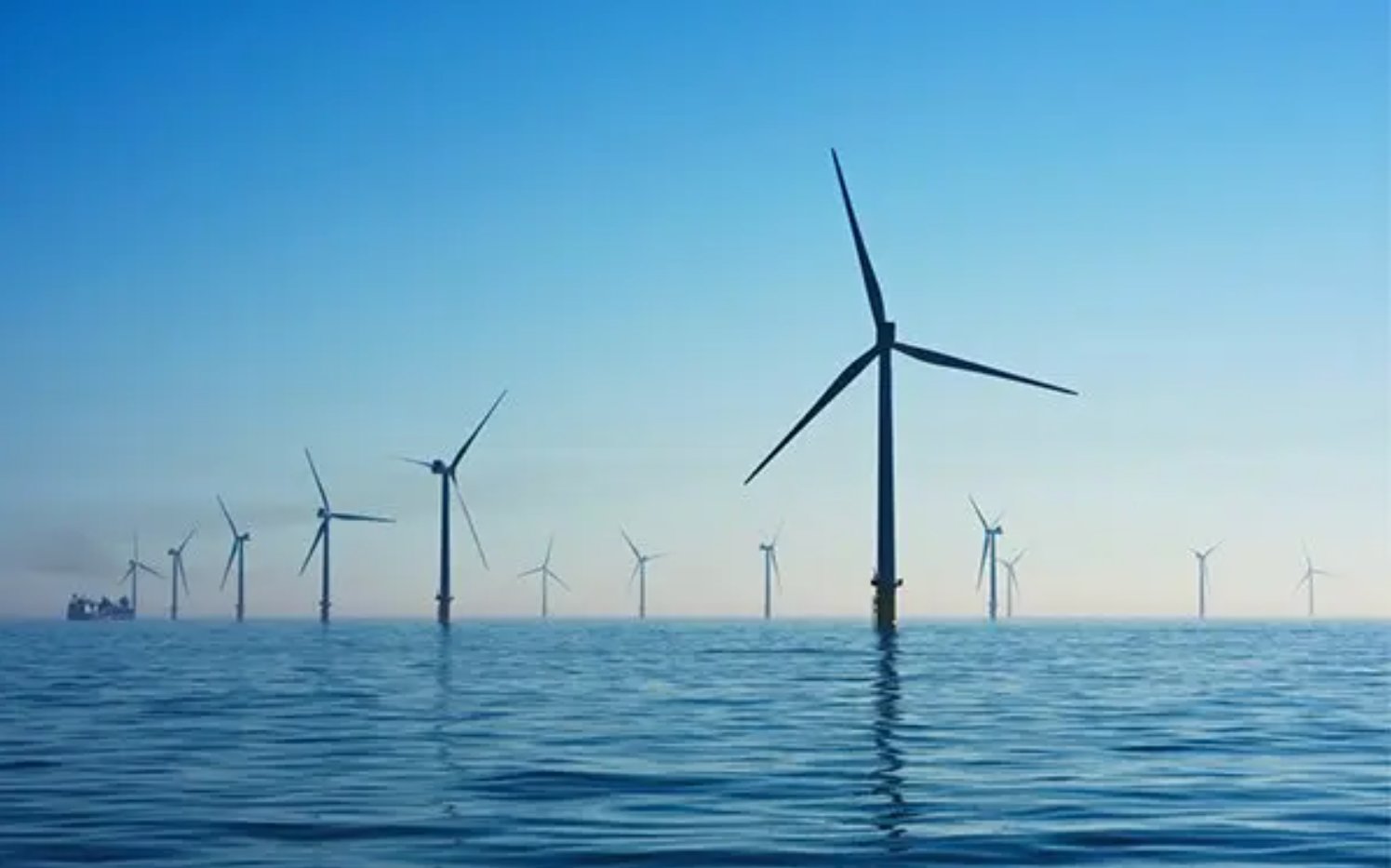The photograph captures a serene ocean scene at either sunrise or sunset, evidenced by the hues of the sky transitioning from deep blue to a soft pink near the horizon. The calm, pristine blue water gently ripples beneath a sprawling wind farm. A total of 13 wind turbines, characterized by their sleek, three-pointed blades, rise gracefully from the water, arranged in linear rows. The turbines, likely a gray or silver shade, cast subtle reflections in the tranquil sea. In the far left background of the image, a boat or possibly an oil rig or tanker is faintly visible, adding a touch of intrigue to the peaceful setting. The image, dominated by the vast expanse of water and sky, is a captivating portrayal of renewable energy harnessed amidst natural beauty.